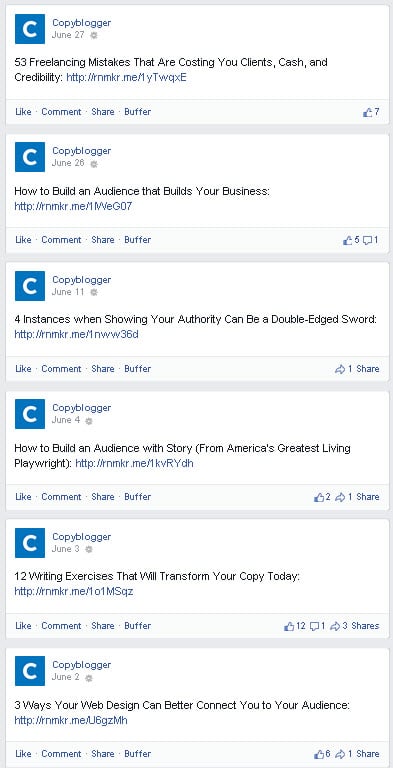The image is a screenshot showcasing a Copyblogger article published on June 27 titled, "53 Freelancing Mistakes That Are Costing You Clients, Cash, and Credibility." The post includes interactive buttons for liking, commenting, sharing, and buffering. Below this article, there are three additional posts listed:

1. "Copyblogger, June 26: How to Build an Audience That Builds Your Business. Four Instances When Showing Your Authority Can Be a Double-Edged Sword."
2. "How to Build an Audience with Story from America's Greatest Living Playwright."
3. "12 Writing Exercises That Will Transform Your Copy Today. Three Ways Your Web Design Can Better Connect You to Your Audience."

A blue-colored link is situated at the bottom of the image. The post has received one share and six likes.